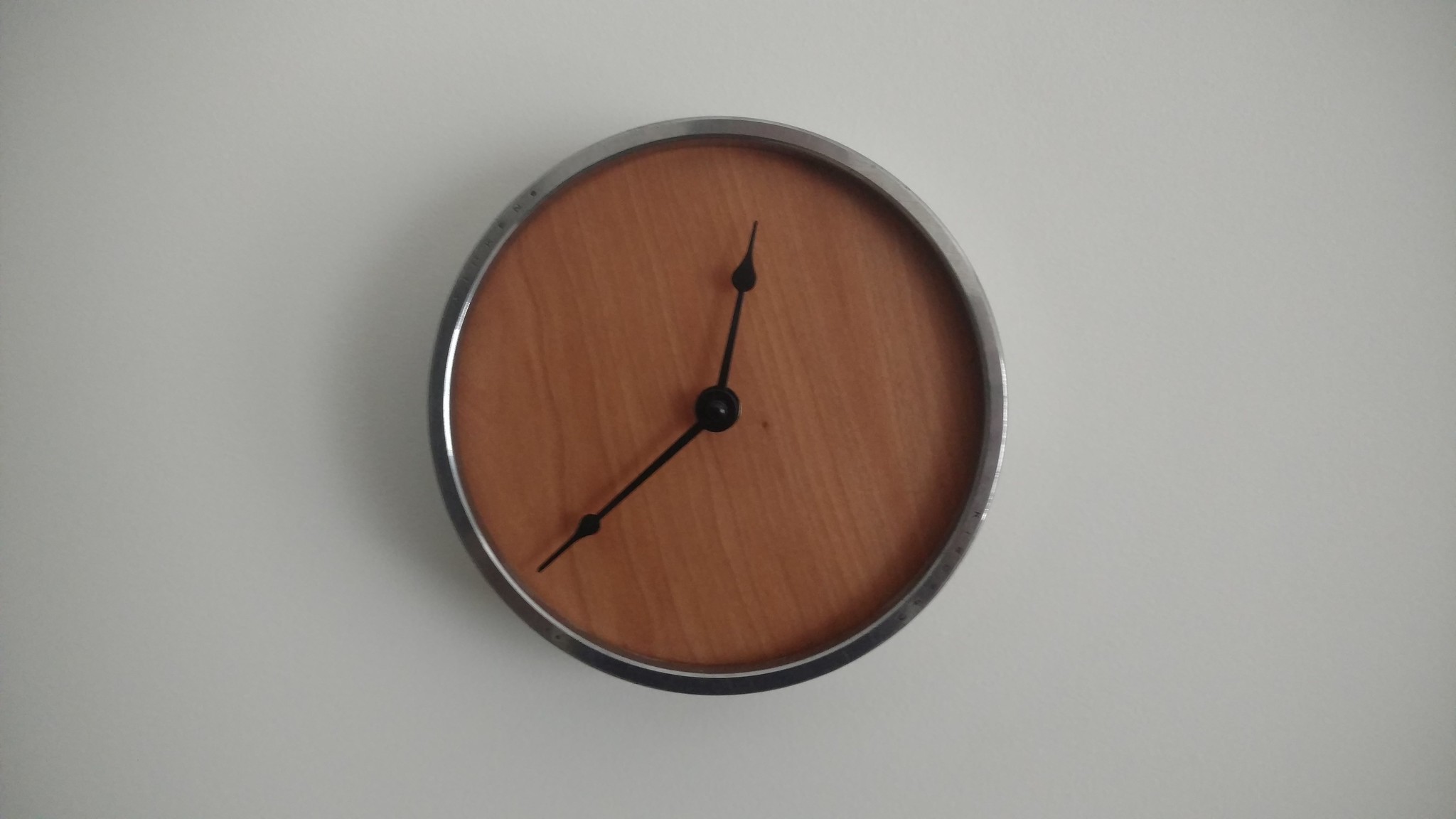This rectangular image features a centrally placed circular clock against a light gray background. The clock, highlighted by its silver border, has a rich, brown face with a wooden pattern. Its design is minimalist, lacking numerical markers, and instead only featuring black hands. A subtle shadow on the left side adds depth to the scene.